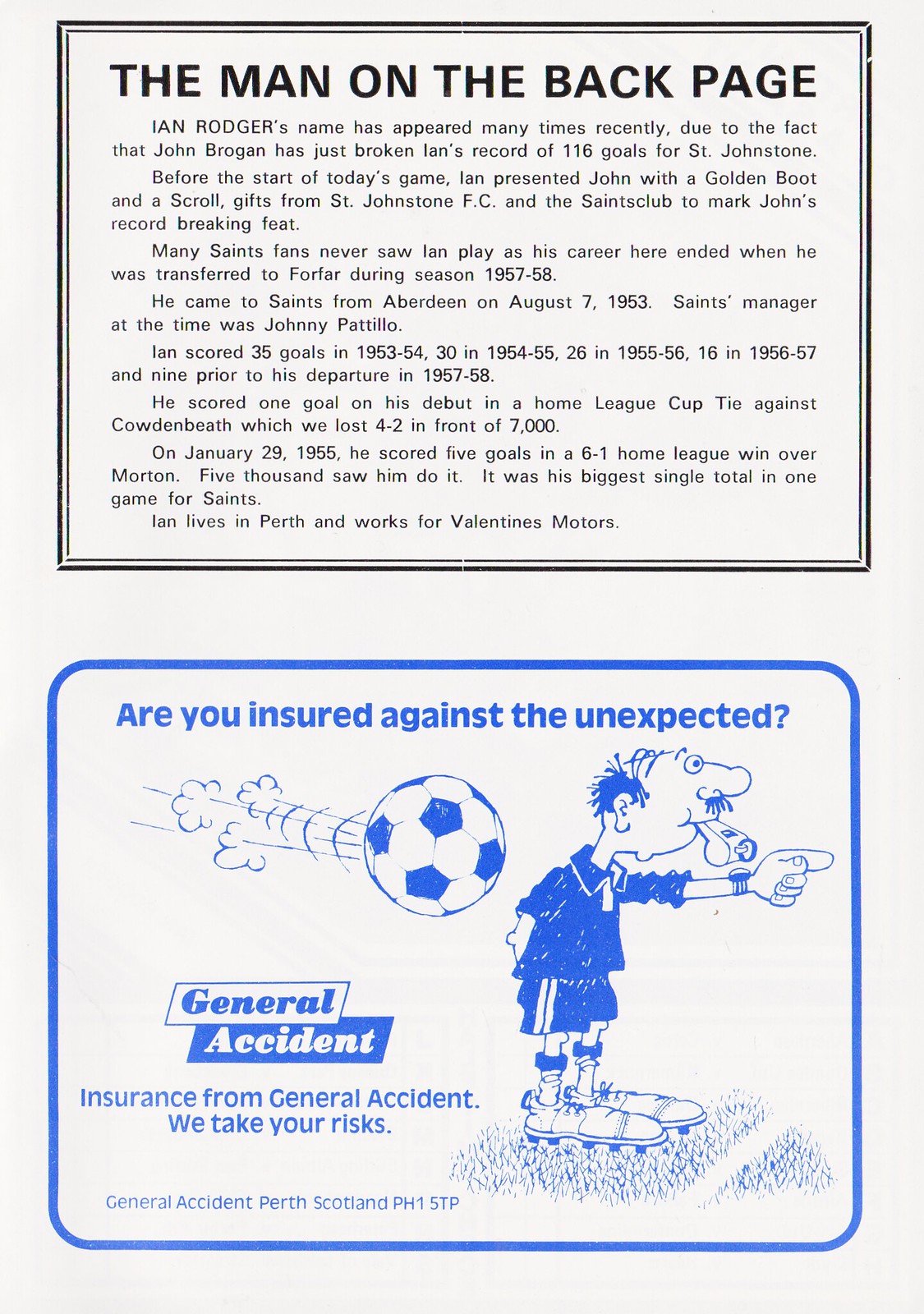This vintage advertisement, potentially from a 1950s or 1960s newspaper, brochure, magazine, or book, is split into two distinct sections. At the top, under the heading "The Man on the Back Page," the ad focuses on Ian Rogers, whose name has recently been in the spotlight because John Brogan has surpassed his record of 116 goals for St. Johnstone. Prior to the start of a recent game, Ian presented John with a golden boot and a scroll, gifts from St. Johnstone FC and the Saints Club, to honor John's accomplishment. This section is filled with additional text, including more detailed information, dates, goal points, and a brief biography of Ian Rogers.

The bottom section features another advertisement with the headline "Are you insured against the unexpected?" It includes a cartoon illustration of a referee about to be struck from behind by a soccer ball. The referee is depicted blowing a whistle. The caption at the bottom of the illustration reads, "General Accident – Insurance from General Accident, We take your risks."